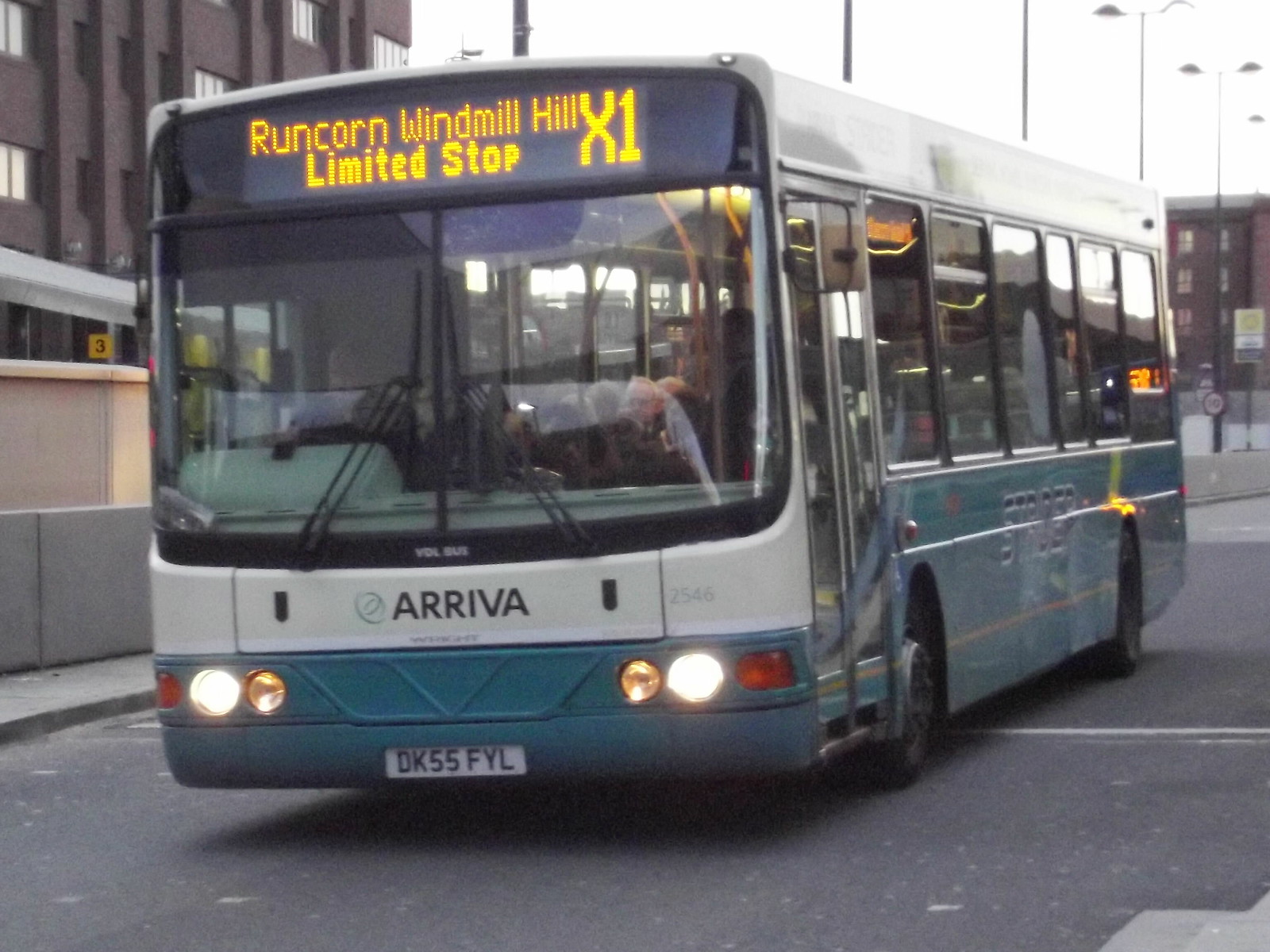An Arriva metro bus is seen driving along a city street, flanked by tall buildings on either side. The bus features a large, modern windshield, largely obfuscating the view of its interior, with just a faint reflection of the driver visible as he holds the steering wheel. The electronic reader board above the windshield displays "Runcorn Windmill Hill, Limited Stop, X1" in yellow. The bus appears to be a 30-seater based on its length and the window arrangements along the side. Its flat-faced front showcases the headlights and a low-mounted license plate underneath the prominent Arriva logo. The bus is primarily painted in gray with teal accents. The vehicle is navigating an asphalt street under clear street lights.